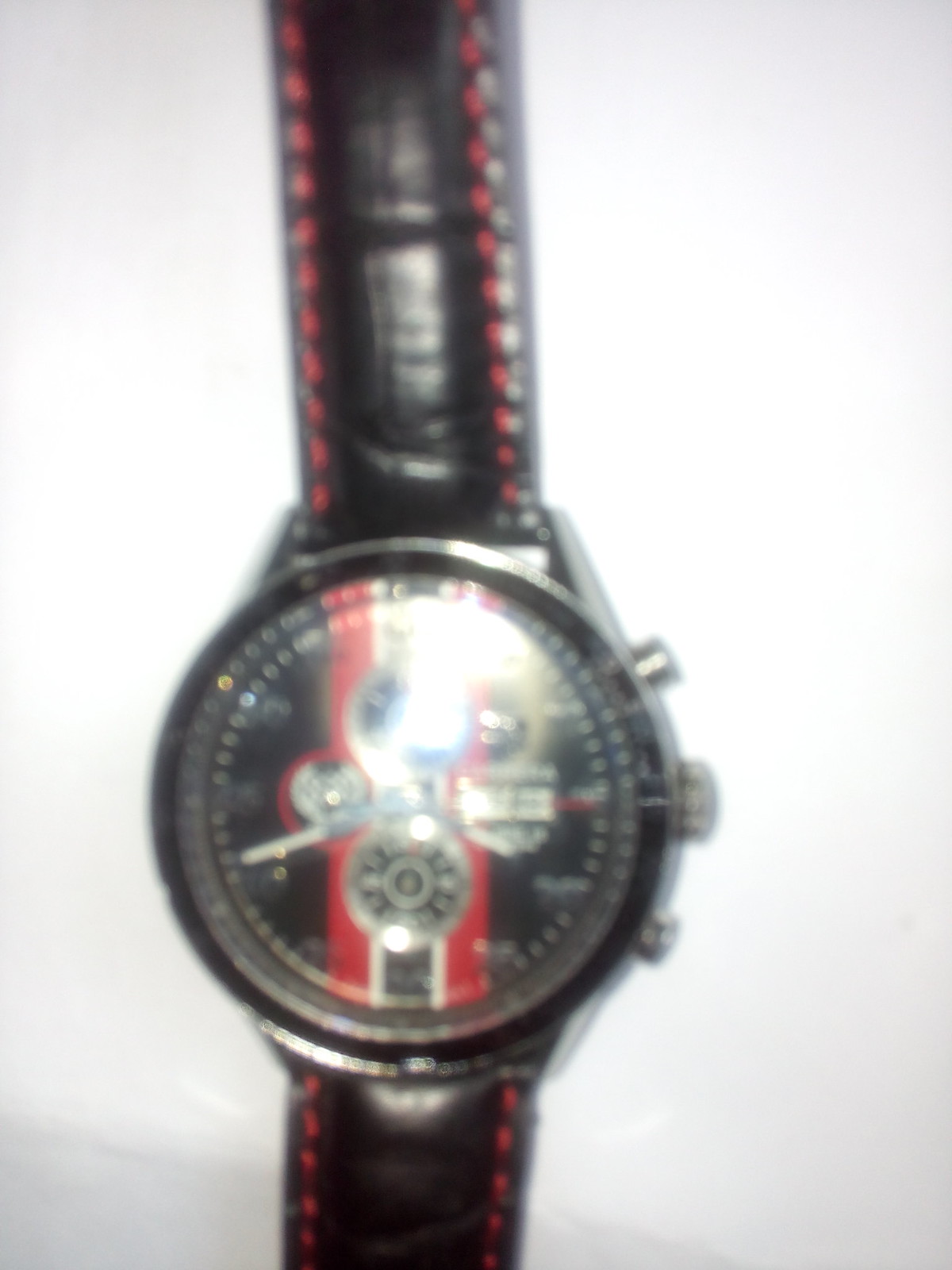This is a vertically aligned, blurry close-up photograph of a wristwatch displayed on a pure white background, possibly a table or a piece of paper, illuminated by a bright camera flash. The watch features a black leather band with red stitching along both edges, spanning from the top to the bottom of the image. The watch face is predominantly black with a bold red stripe running vertically from the 12 o'clock to the 6 o'clock position, intersected by silver hands and arranged gears in the center. The right side of the watch displays three gear switches, presumably to set the time and date. The flash reflection creates a white shine across the watch face and the glossy, well-worn leather band, further distorting the image details.